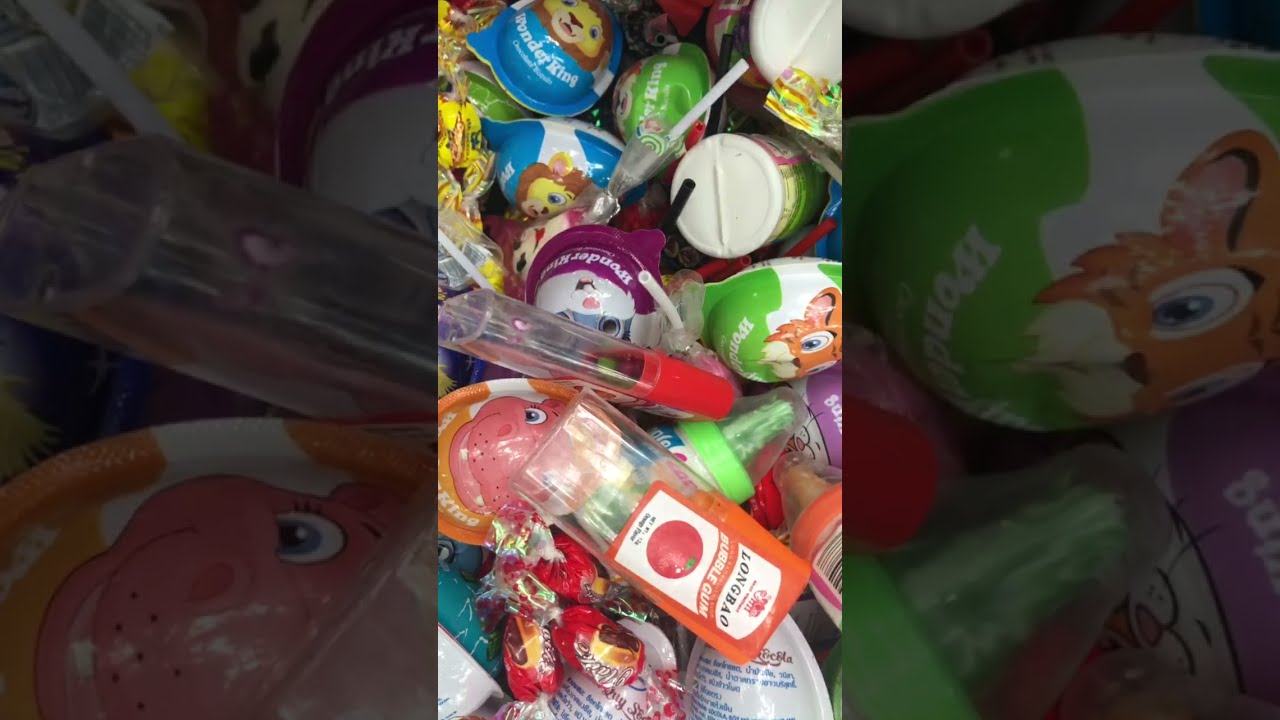The image captures a cluttered assortment of candies and small toys, likely aimed at children, displayed in a colorful yet chaotic manner. The photo itself seems to be a snapshot taken from a cell phone, evident by the darkened left and right areas framing the central portion of the image. Dominating the scene are various candies wrapped in vibrant packaging, including round chocolate eggs adorned with whimsical designs of animals such as lions, tigers, hippos, and rabbits. Among the mix, certain items stand out, like a "Wonder King" egg, reminiscent of a Kinder Surprise, and a Long Bell Bubble Gum wrapper featuring what appears to be a tomato illustration.

Scattered within the pile are hard candies encased in plastic twist wraps, primarily red, along with multiple lollipops including one stylized with a clown face. A notable observation is the predominance of egg-shaped candies over other types. Despite numerous text inscriptions visible on the packaging, they are largely indecipherable, suggesting non-English labeling, adding a layer of mystery to the assortment. The variety of treats in blue, green, orange, and purple wrappings, each with distinctive cartoonish faces, underline the playful, child-friendly theme of the collection.